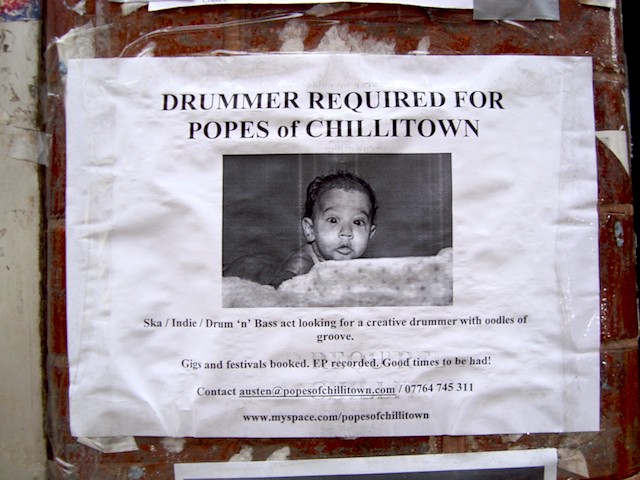This picture shows a flyer seeking a drummer for the band Popes of Chillytown. The flyer, made of white computer paper, is taped to a dark red surface, possibly a trash can or a brick wall, and reinforced with clear tape. The title, "Drummer Required for Popes of Chillytown," is displayed prominently in large red font at the top. Below the title, a black-and-white photo of an African American baby with dark curly hair, possibly under a year old, is featured; the baby appears to be lying on its stomach, perhaps in a crib or on a blanket. Under the photo, the text describes the band as a "Ska/Indie/Drum and Bass" act seeking a creative drummer "with oodles of groove" for gigs and festivals that are already booked, and an EP that has been recorded. The flyer promises "good times to be had!" It provides contact information for Austin, spelled A-U-S-T-E-N, with an email address at popesofchillytown.com and a phone number, 077-647-45311. At the bottom, there is a MySpace link: www.myspace.com/popesofchillytown.